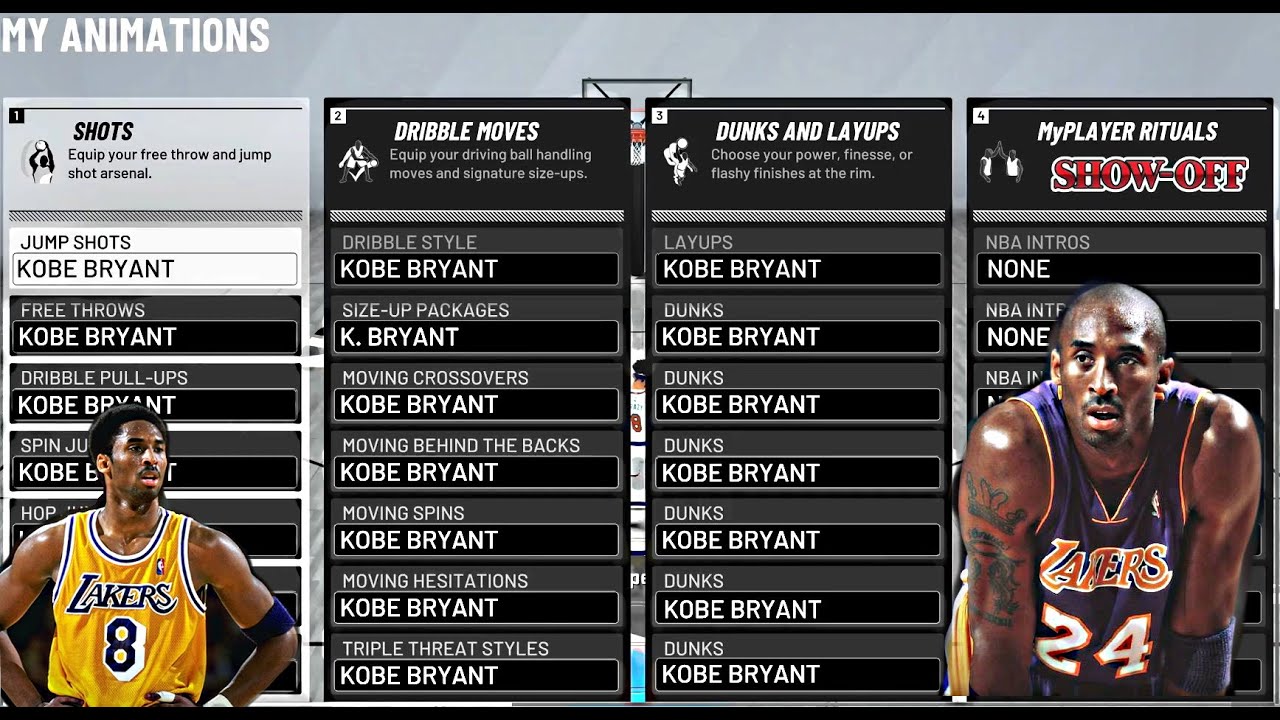The image displays various basketball moves and skills, primarily featuring Kobe Bryant, on a light purple background. The image is framed with a heavy black line at the top, a light purple line along the left side, and a heavy black line at the bottom.

- **Top Section:**  
  The top section starts with a "My Animations" title in white font against the purple background. Below this is a small black box labeled "1" followed by the text "Shots: Equip Your Free Throw and Jump Shot Arsenal." Two white boxes underneath display "Jump Shots" and "Kobe Bryant."

- **Skill Details:**  
  Below the initial description are several black boxes featuring skills associated with Kobe Bryant:
  - **Free Throws: Kobe Bryant**
  - **Dribble Pull-ups: Kobe Bryant**
  - **Spin Jumps: Kobe Bryant**

- **Middle Section:**  
  The second main section has a black box with a "2" and the heading "Dribble Moves: Equip Your Driving Ball Handling Moves." This is followed by "Signature Size-ups" and a variety of dribbling styles featuring Kobe Bryant:
  - **Dribble Style: Kobe**
  - **Size-up Packages: Kobe**
  - **Moving Crossovers: Kobe**
  - **Moving Behind the Backs: Kobe**
  - **Moving Spins: Kobe**
  - **Moving Hesitations: Kobe**
  - **Triple Threat Styles: Kobe**

- **Third Section:**  
  The third section features a black box labeled "3" and focuses on "Dunks and Layups: Choose Your Power, Fitness, or Flashy Finishes at the Rim." Further down are multiple examples of Kobe's finishing moves:
  - **Layups**
  - **Dunks**
  - **Dunks**
  - **Dunks**
  - **Dunks**
  - **Dunks** (all variations featuring Kobe Bryant)

- **Bottom Section:**  
  The final section has a white box and line labeled "My Player Rituals," followed by the text "Show Off" in red. Additional details include:
  - **NBE: Nitros (None)**
  - An image of the Lakers' number "24," representing Kobe Bryant.

This comprehensive description encapsulates all elements of the depicted skills, providing a clear and structured breakdown of the content featuring Kobe Bryant's animations and moves.